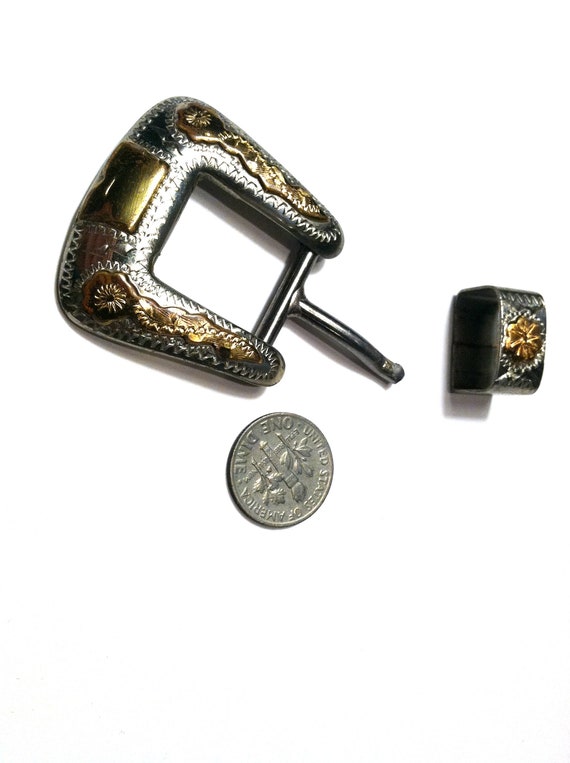The image depicts a detailed close-up of a silver belt buckle, elegantly adorned with brass plant designs and a rectangular gold centerpiece. The buckle has a letter 'C' shape connected by a thin metal bar, possibly meant to hook into a belt hole. To its right, within the vertical frame, there is another smaller, similarly decorated hollow piece. Below the buckle, there's a dime placed with its tails side facing up, inscribed with "United States of America, One Dime," and featuring the torch and plant imagery typical of the coin. The objects' colors include silver, gold, brass, black, and white, with the photograph styled as a product image for showcasing the belt buckle and its details.